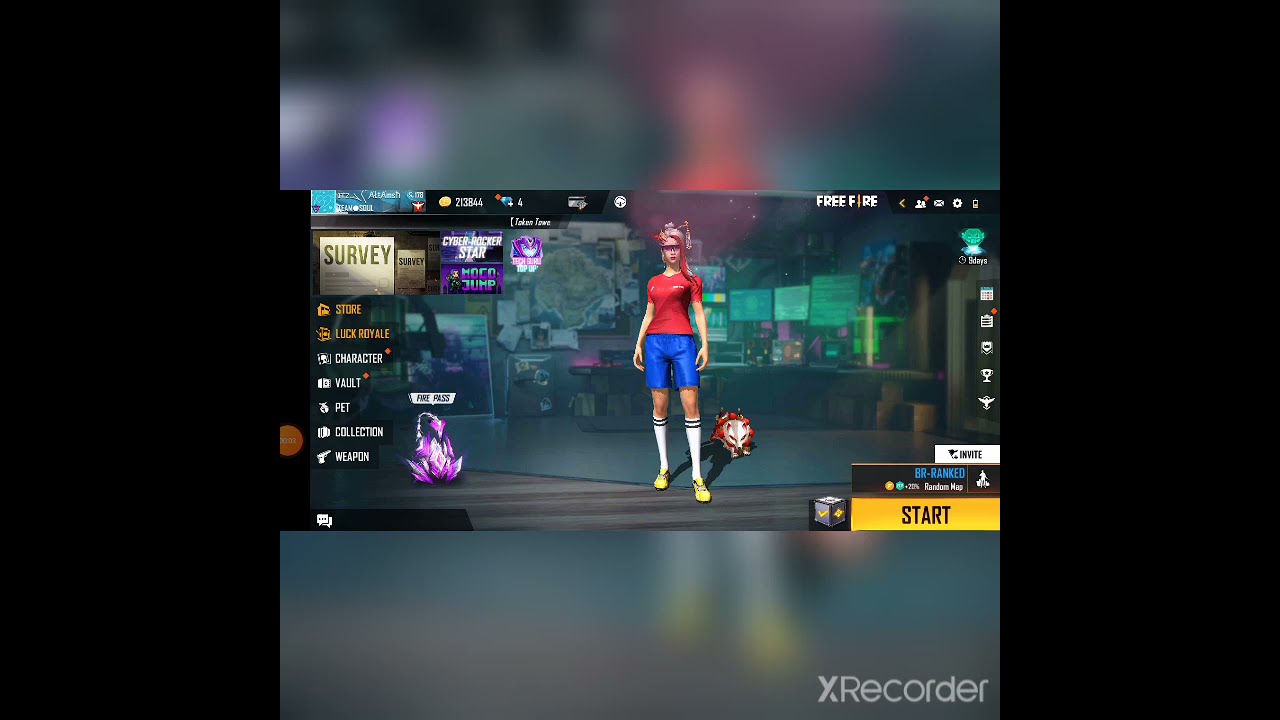In this video game screenshot, a central female character is featured, presenting an athletic and vibrant appearance. She is a white girl with shoulder-length blonde hair accented with red streaks, and she is adorned with a butterfly in her hair. She wears rose-colored sunglasses and a tight, red, short-sleeved compression shirt, paired with royal blue shorts. Completing her outfit are knee-high white socks with two black stripes at the top and yellow sneakers. To her left, the game interface displays a menu with various options including 'Character Vault', 'Pet Collection', 'Weapons', 'Store', and 'Luck Royale'. Behind her, a possum-like creature in a red dress is positioned near the ground. The background is a blurred cityscape, adding depth to the image. The bottom right corner of the screen shows the "Start" button, indicating the beginning of gameplay, and the watermark ‘X-Recorder’ suggests the image is a recording. At the top, there is a display of in-game currency, with the character having over 200,000 gold coins.